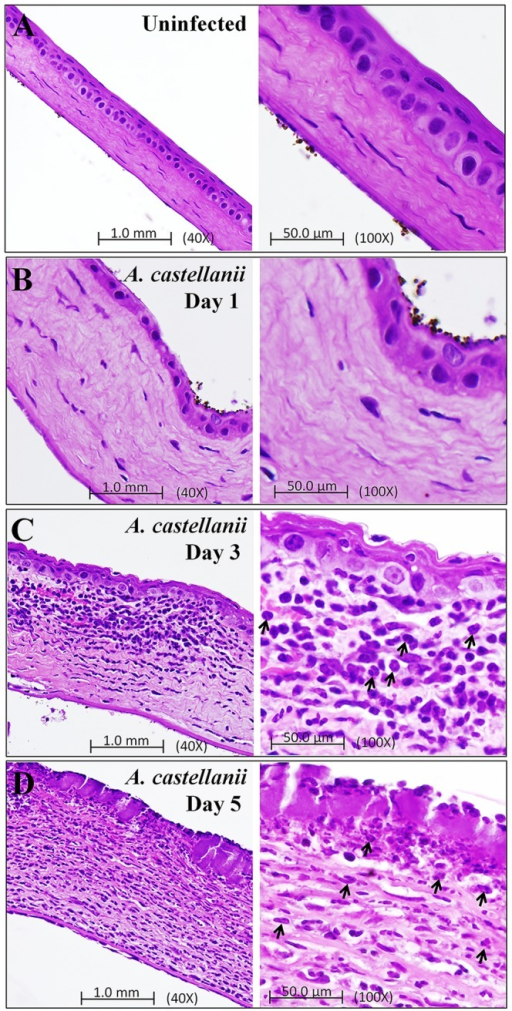This image set consists of eight microscope photos arranged in two columns. Each photo's background is white, and the objects in the images are purple strands. The top left image, labeled "A" and identified as "uninfected," displays a thin, straight purple strand at two different magnifications: 1.0 millimeters at 40x and 50.0 micrometers at 100x. Below it, image "B" shows "A Castellani Day One," revealing a purple band that is now wavier and more irregular, with two pictures at similar magnifications. Image "C," labeled "A Castellani Day Three," features a strand that is less wavy but populated with numerous dark purple dots. Finally, image "D" at the bottom, labeled "A Castellani Day Five," depicts the strand covered with even more dark purple dots, almost filling the original lighter purple area, with another zoomed-in image for detailed observation. The right column consistently shows a more magnified close-up of the corresponding left image, emphasizing increased detail and bacterial activity over time, marked by spreading holes and darker areas.